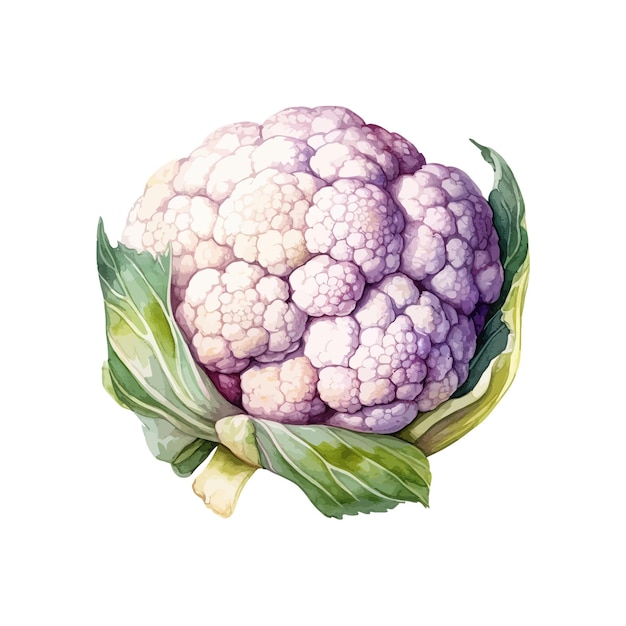In this illustration, we see a detailed depiction of a cauliflower plant with an unusual coloration. The central focus is the cauliflower itself, which is characterized by its multi-lobed, bulbous form. Unlike the typical white cauliflower seen in grocery stores, this cauliflower exhibits a unique blend of purplish and cream hues. Surrounding the cauliflower are several veined leaves in various shades of green, from light to dark, cradling it from the bottom left and right. The leaves, complete with white veins, add a realistic touch to the plant's overall structure. The background of the illustration is plain white, emphasizing the cauliflower and its leaves. The artist or purpose of the illustration remains unidentified, and no additional contextual information or people are included in the image.